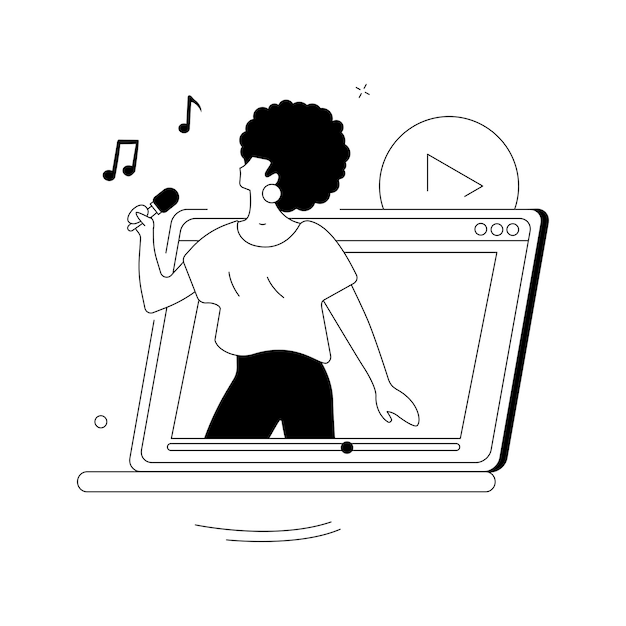The image is a simplistic black and white graphic with a distinct 70s disco vibe, featuring a figure of a woman emerging from what appears to be a computer or tablet screen. She has an afro hairstyle and wears a short sleeve white shirt paired with dark pants. Her face is featureless, resembling a cartoon silhouette, and she's accessorized with large round earrings. Holding a microphone in her right hand, which is slightly bent towards her mouth, she looks like she's singing, highlighted by music notes near her face and the microphone. A play button symbol, depicted as a circle with a right-facing triangle, is positioned at the top of the screen backdrop, enhancing the audio-visual theme of the illustration.